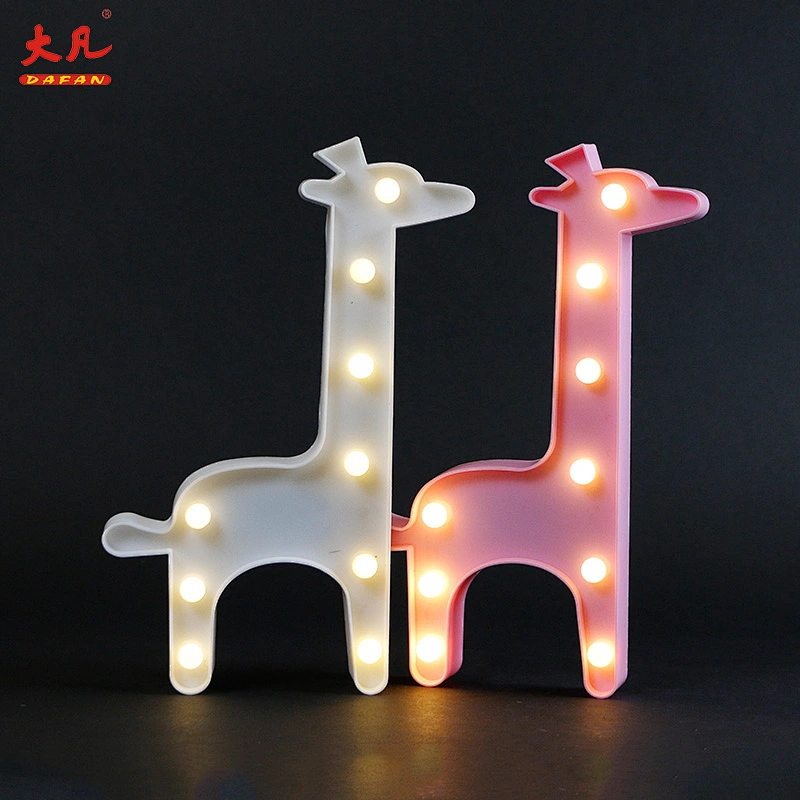The photograph features two simple plastic giraffe figurines designed as backward H shapes. The giraffes have elongated necks forming the top of the H, while the body forms the loop, and a tail extends from the rump. Each giraffe is embedded with nine light bulbs: one row running from the head down to one foot and another from the rump to the other foot. The white giraffe stands on the left, and the pink, or mauve, giraffe is on the right. Both giraffes have small lit horns and ears. In the top left corner of the black canvas background, there are Asian characters along with the text "Daffan" in English. The lights in the figurines give them a glowing appearance, making them suitable as decorative pieces.